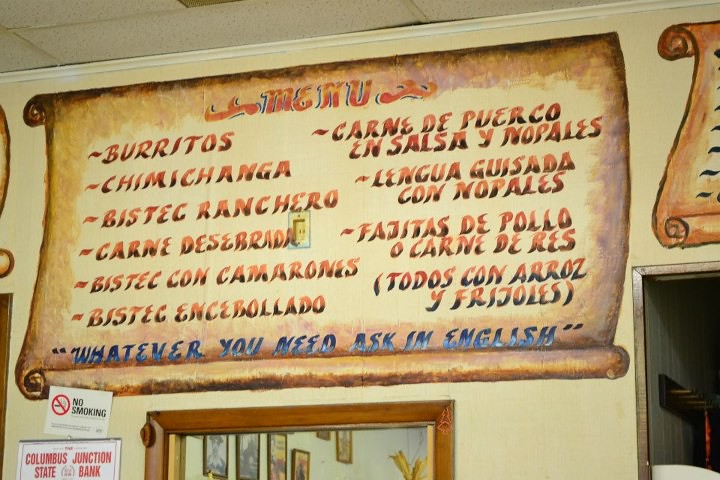In the image, there is a vivid painting on a wall, designed to resemble a traditional scroll, which serves as a menu likely from a Mexican restaurant. The vibrant painting features the word “Menu” prominently at the top, with items such as burritos, chimichangas, and fajitas listed below. The menu text is artistically rendered in shades of red and blue, giving it a festive and eye-catching appearance. Further down the scroll, it advises in blue ink, "Whatever you need, ask in English." Adjacent to the painted menu are two white placards affixed to the wall. One placard, written in black ink, clearly states "No Smoking." The second placard, inscribed in red ink, reads "Columbia’s Junction State Bank." The overall scene suggests a cozy and thoughtfully decorated dining area where specific messages guide patrons effectively.